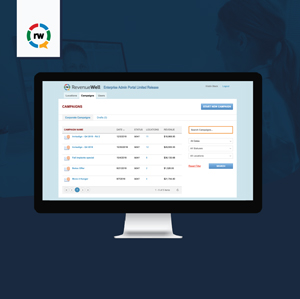The image features a blue background with a partial view of a woman on the right. She has her hair tied in a ponytail and is facing away from the camera, looking towards a screen on the left. The screen displays a faint image of a man's face, but it is largely obscured by another image in the foreground.

In the foreground, there's a prominent monitor with a thick black bezel resembling an Apple monitor. The screen displays a light blue page with faint, small text, likely reading something similar to "river plus well." The resolution of the text is poor, making it difficult to decipher. The page appears to feature a white chart with tabs at the top, marked by prominent red headlines.

On the right side of the monitor's display, there are yellow and blue links, blue buttons, and an area framed by an orange border. The monitor itself is mounted on a silver stand. At the top left corner of the screen, there's a white area with a speech bubble icon in red, blue, and green colors, containing the initials "NW" in black.